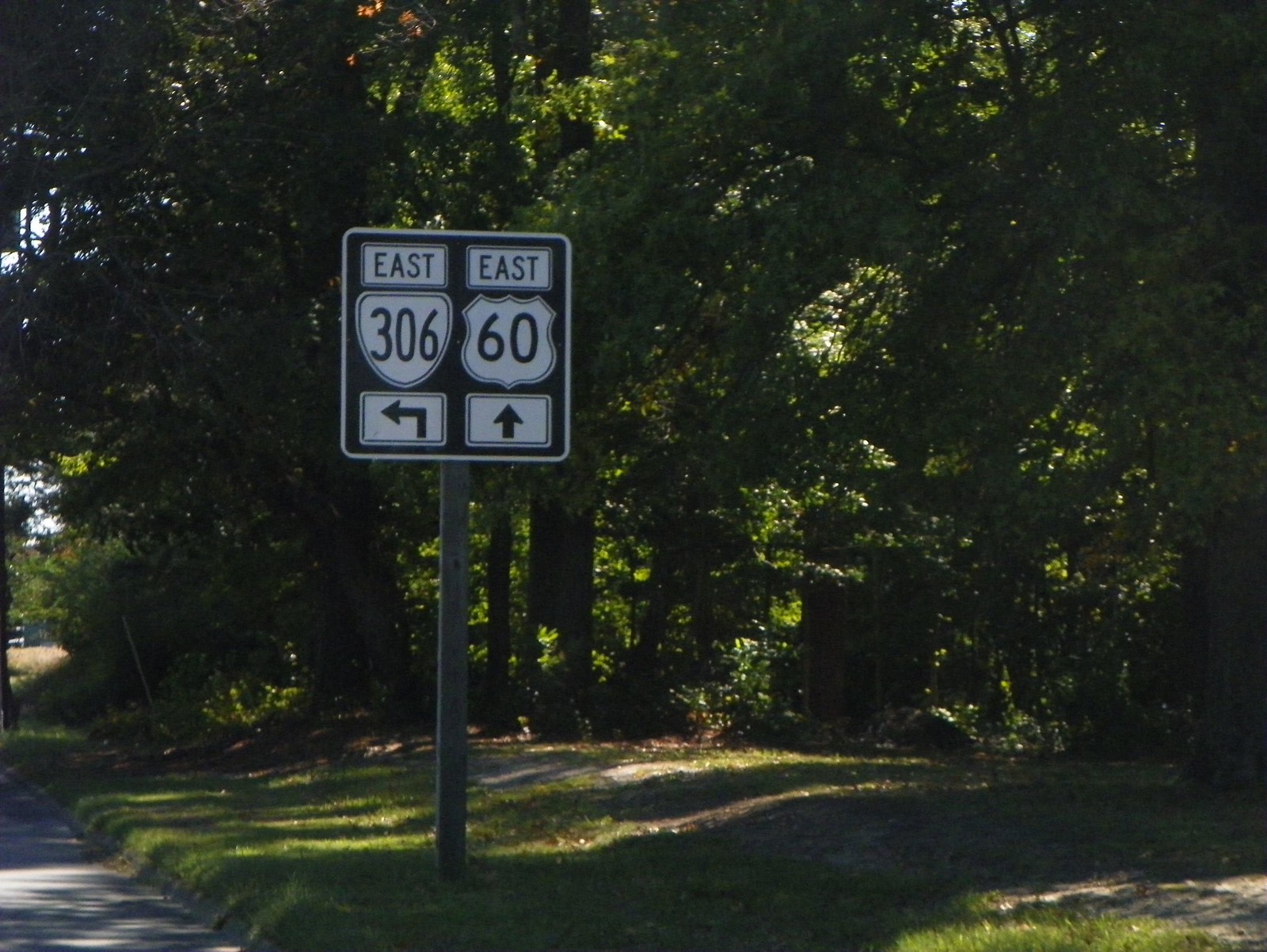The image depicts a serene path nestled within a neighborhood, serving as an alternative route to bypass the main highway. The path is unpaved, its dirt surface showing signs of frequent use, possibly by local children and residents with four-wheelers. Flanking the path is a dense array of trees, their branches creating a natural canopy and adding to the tranquil atmosphere.

In the distance, a two-lane road becomes visible, partly obscured by the trees. A prominent street sign stands at the road's edge, perched on a wooden block. The sign is black and white, featuring a rectangle with "EAST" written in bold black letters on a white background. Directly below, there is an almost upside-down triangle shape displaying the number "306." An arrow pointing left is situated within another rectangle, indicating a left turn. Additionally, another section of the sign directs travelers to continue straight ahead for route "EAST 60."

Ahead on the road, a car approaches, emphasizing the path's connection to a larger network of routes and the community through which it weaves.